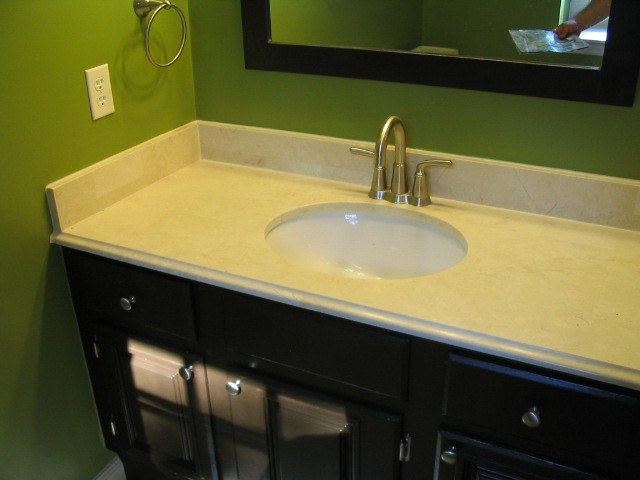A detailed caption for the bathroom vanity image could be: 

"The bathroom features a vanity with a dark wooden cabinetry that consists of several drawers and dual doors, each equipped with a sleek silver knob. Atop the cabinet is a white imitation marble surface with a smooth oval cutout housing a white sink. The surface is accompanied by a matching white backsplash approximately five inches in height. The surrounding walls are painted a soothing sea green, complementing the vanity's design. On the left wall, there's a white power outlet and a silver towel ring, currently empty. Above the vanity, a large rectangular mirror with a dark wooden frame that matches the cabinetry extends upward, though only the bottom portion is visible in the image. The sink is fitted with a dual-handle faucet, featuring separate controls for hot and cold water, and a gooseneck spigot that allows for adjustable water flow direction. The vanity top is uncluttered and devoid of any items."